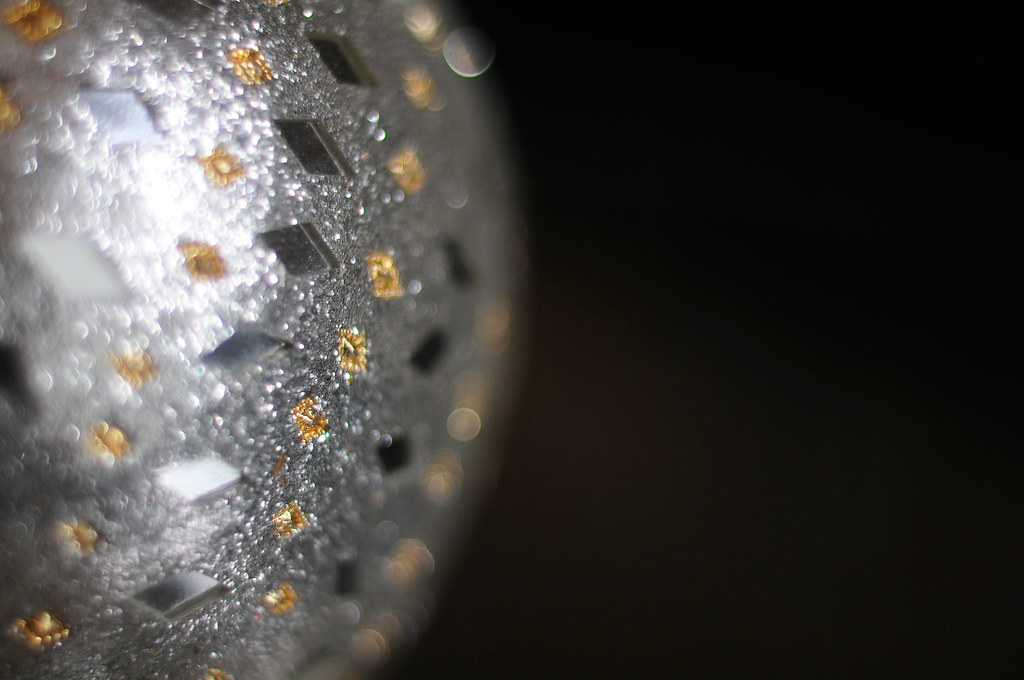In the left half of the image, against a pitch-black background, a close-up of a round, glittery decorative item prominently stands out. The sphere, possibly a Christmas decoration, exhibits a main color palette of silver and gold, adorned with intricate details. The silver area is speckled with small, gold-diamond-like particles arranged in a linear fashion, imparting an opulent sparkle. Interspersed among these glittery elements are black, diamond-shaped pieces that contribute to the jewel-like texture and appearance of the object. The edges where the silver meets the background are blurred, creating a soft transition into the surrounding darkness. The central area of the sphere also features white dots, adding to the textured and dynamic surface. The overall composition juxtaposes the glimmering ornament against a stark, dark void, highlighting its festive and luxurious design.